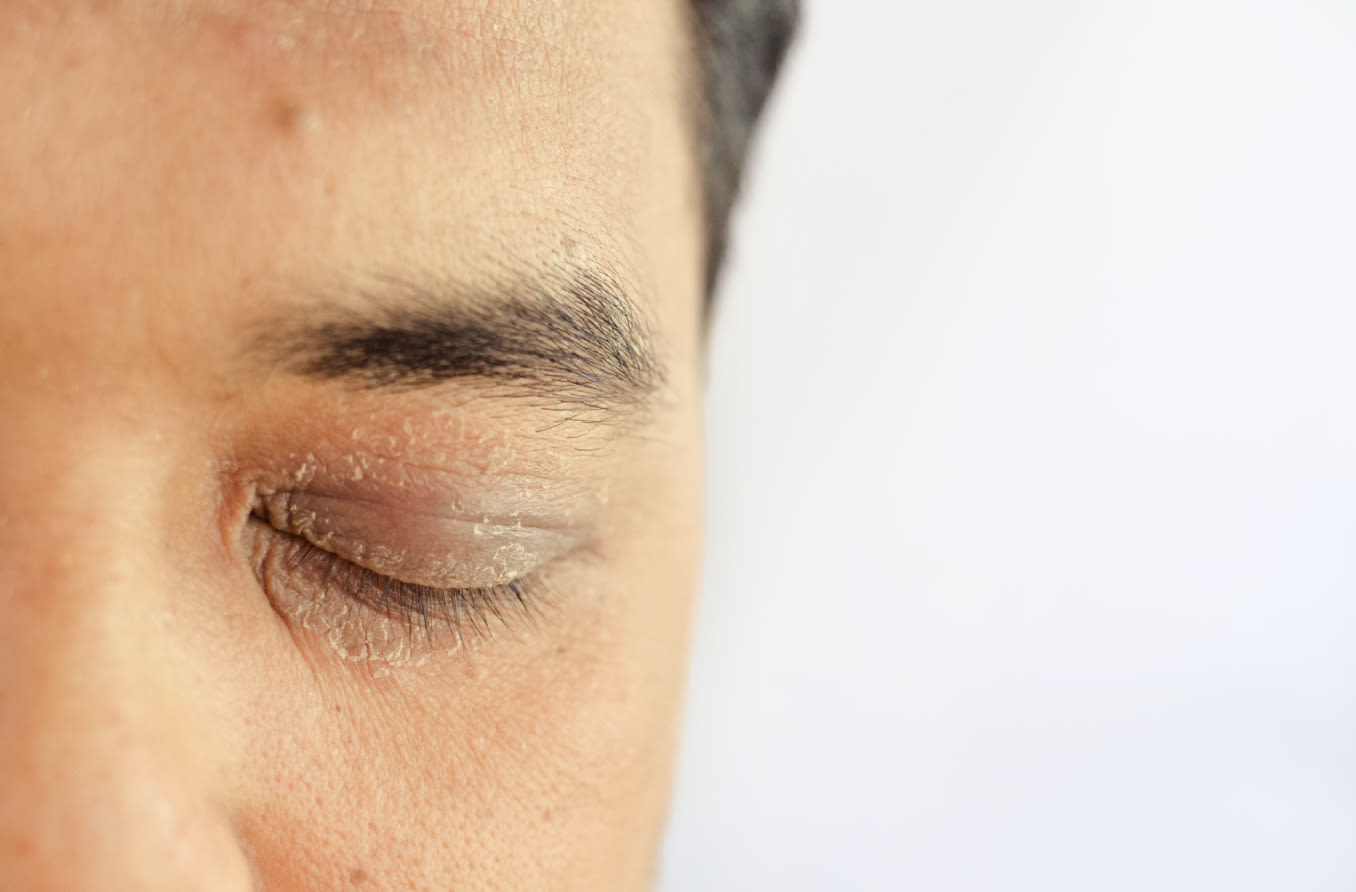The photograph is a detailed close-up of the left side of a man's face, zoomed in to primarily showcase his eye and the immediate surrounding area. His eye is closed, revealing darker colored eyelids adorned with black eyelashes. His eyebrow is also black, contrasting with his light-colored, Caucasian skin. The image captures short, black to brown hair, with some visible at the edge of the frame. Dry, flaky skin is noticeable below and on the eyelid itself, extending slightly to the nearby regions, including some patches on the forehead. Additionally, there are a couple of small bumps or pimples on his forehead. The background is a monochromatic grayish white, occupying the right half of the photograph, which balances the tightly focused and textured detail of the man's eye area. Overall, the composition is horizontally oriented, making the detailed facial features prominent against the plain backdrop.